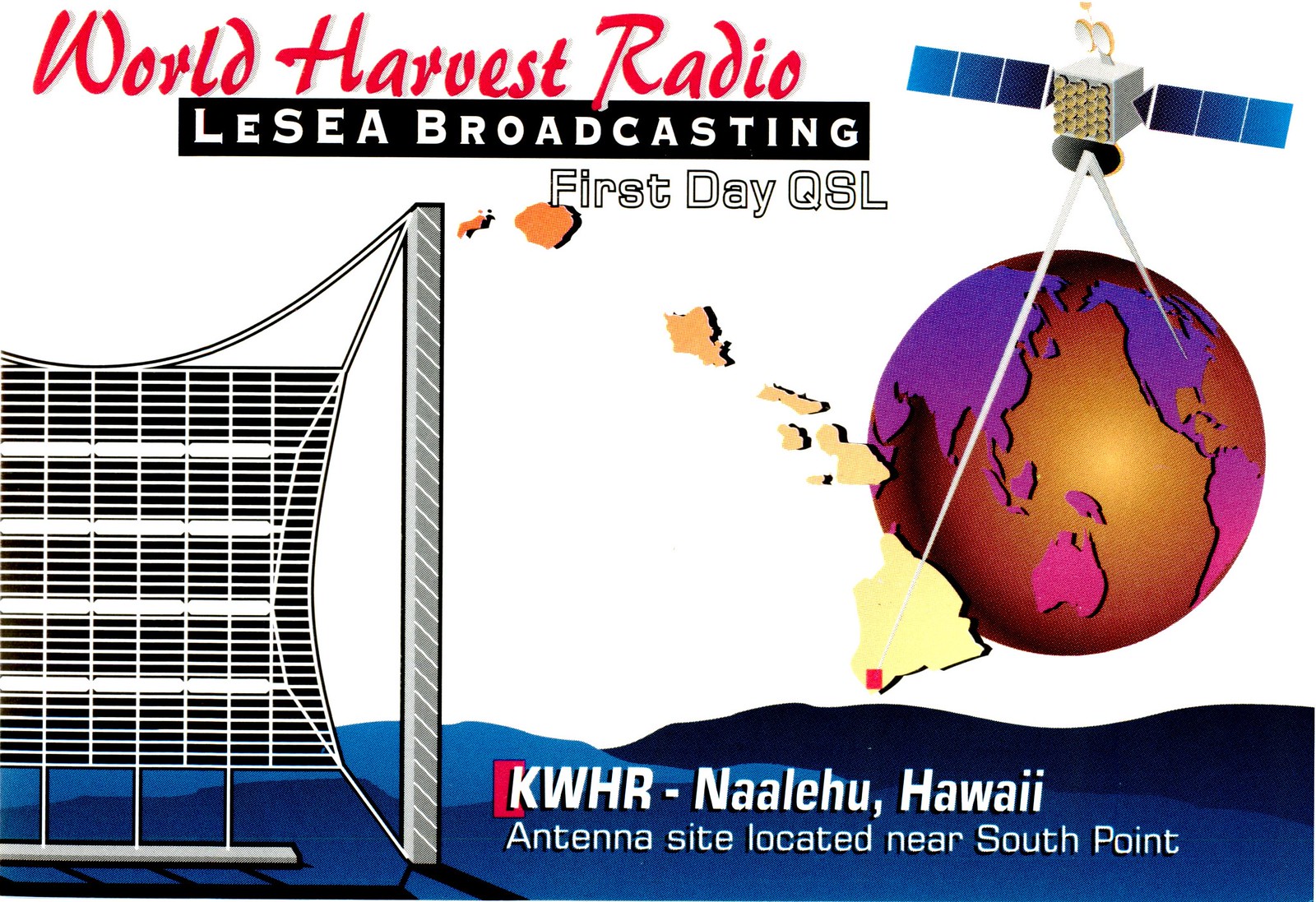The image is a detailed poster titled "World Harvest Radio," printed in bold red letters at the top left-center. Below this title, in a black rectangle with white text, is the phrase "LeSea Broadcasting" followed by "First Day QSL." On the right side, there's a circular globe with a purple background, showcasing the Australian continent in pink. Above the globe, a satellite with flared solar panels emits two rays directed toward the Earth, suggesting a televised image. On the left side of the poster, there's an image resembling a tennis racquet or the silhouette of a grey tower with horizontal stripes. The bottom of the poster features a chain of Hawaiian Islands highlighted in red, with the text "KWHR Lehi, Hawaii" in white letters against a blue mountain outline, and the note "Antenna site located near South Point."